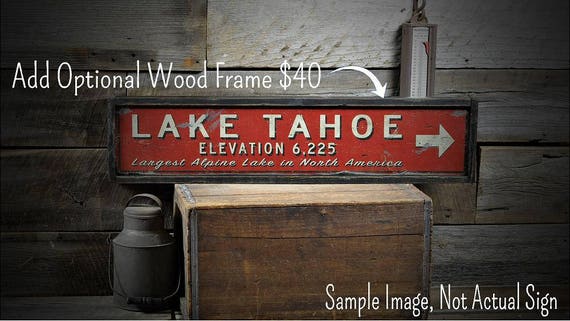In a rustic, dark wood barn setting, this marketing image features a large horizontal wooden sign framed by a dark wood border. The sign, which sits on a light wooden chest with metal edges, has a red painted background with bold white lettering. At the top, "Lake Tahoe" is prominently displayed in all capital letters, followed by a large white arrow pointing to the right. Below this, in smaller bold white text, is the phrase "Elevation 6,225." Further down, in italicized white lettering, it reads "Largest Alpine Lake in North America." Outside the sign's frame, a white arrow points downward with the text "Add Optional Wood Frame $40" above it. On the lower right corner of the image, additional text notes "Sample Image, not Actual Sign." Surrounding the chest and sign, rough-hewn wooden panels create the backdrop, with a vintage dark gray metal milk can placed to the left of the chest and an unidentified cylindrical metal object leaning vertically against the barn wall to the right.